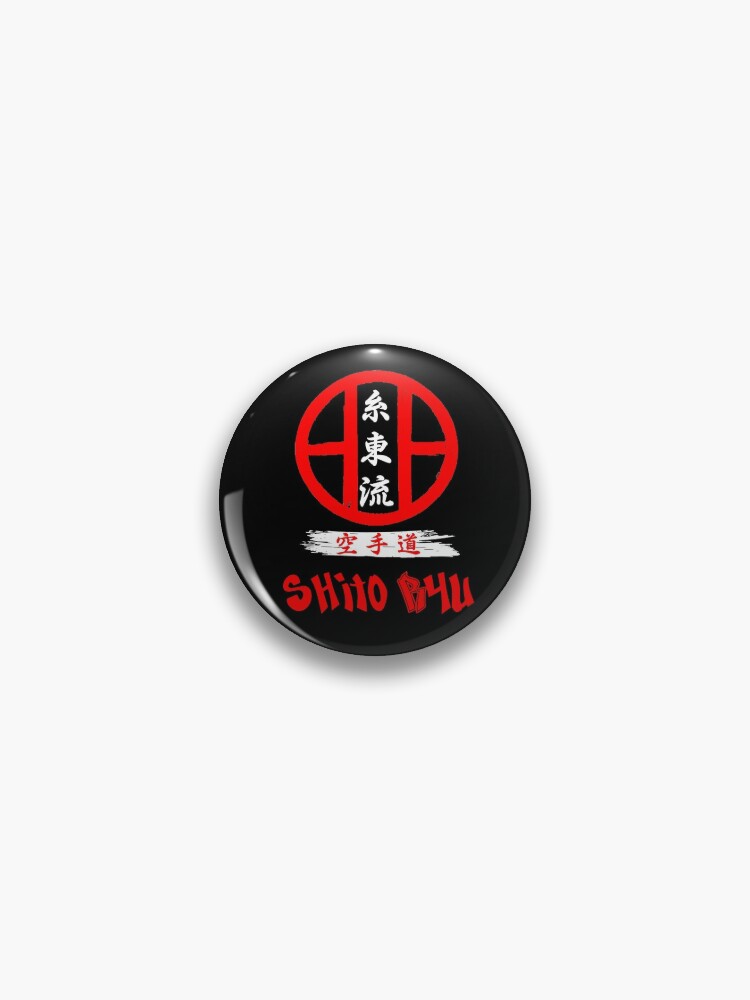The photograph features a small, round button, roughly 1 to 1.5 inches in diameter, designed to be pinned on a jacket or bag. The background is a simple, off-white color with a subtle light gray drop shadow beneath the button, hinting at its shiny surface. The button itself has a base color of black with an intricate design at its center. Dominating the design is a prominent red circle intersected by two vertical and two horizontal red lines. At the core of this red circle, three vertical white kanji characters are prominently displayed. Below the circle, a horizontal white paint stroke contrasts against the black background, overlaid with three red kanji characters. Further below, in red English letters, the text "SHITO B4U" appears. A slight light reflection is noticeable to the left and top of the button, adding a touch of realism to the image.